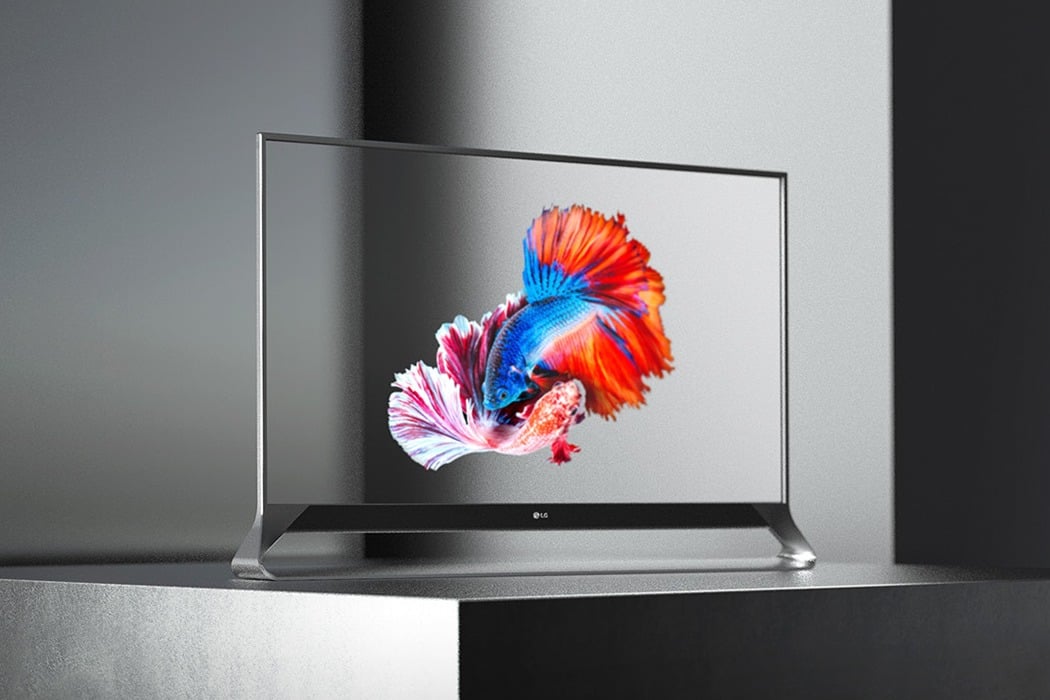This image captures a striking piece of art presented in a minimalist setting. The art features two vividly colored fish entwined in a yin-yang formation, painted on a clear, rectangular glass or acrylic surface. This transparent screen, roughly 14 to 16 inches wide and 12 inches tall, appears to be an LG-branded digital art frame. The image showcases the top fish as blue with a vibrant orange-red tail, while the bottom fish is predominantly pink-orange, adorned with white and reddish accents. The frame is mounted on a sleek, gray pedestal with two legs, which is set upon a gray, possibly metallic or plastic, base. The entire setup rests against a backdrop of black and white, enhancing the vivid colors of the fish. The scene evokes a sense of refined elegance, reminiscent of a museum's minimalist exhibit or a sophisticated modern home.